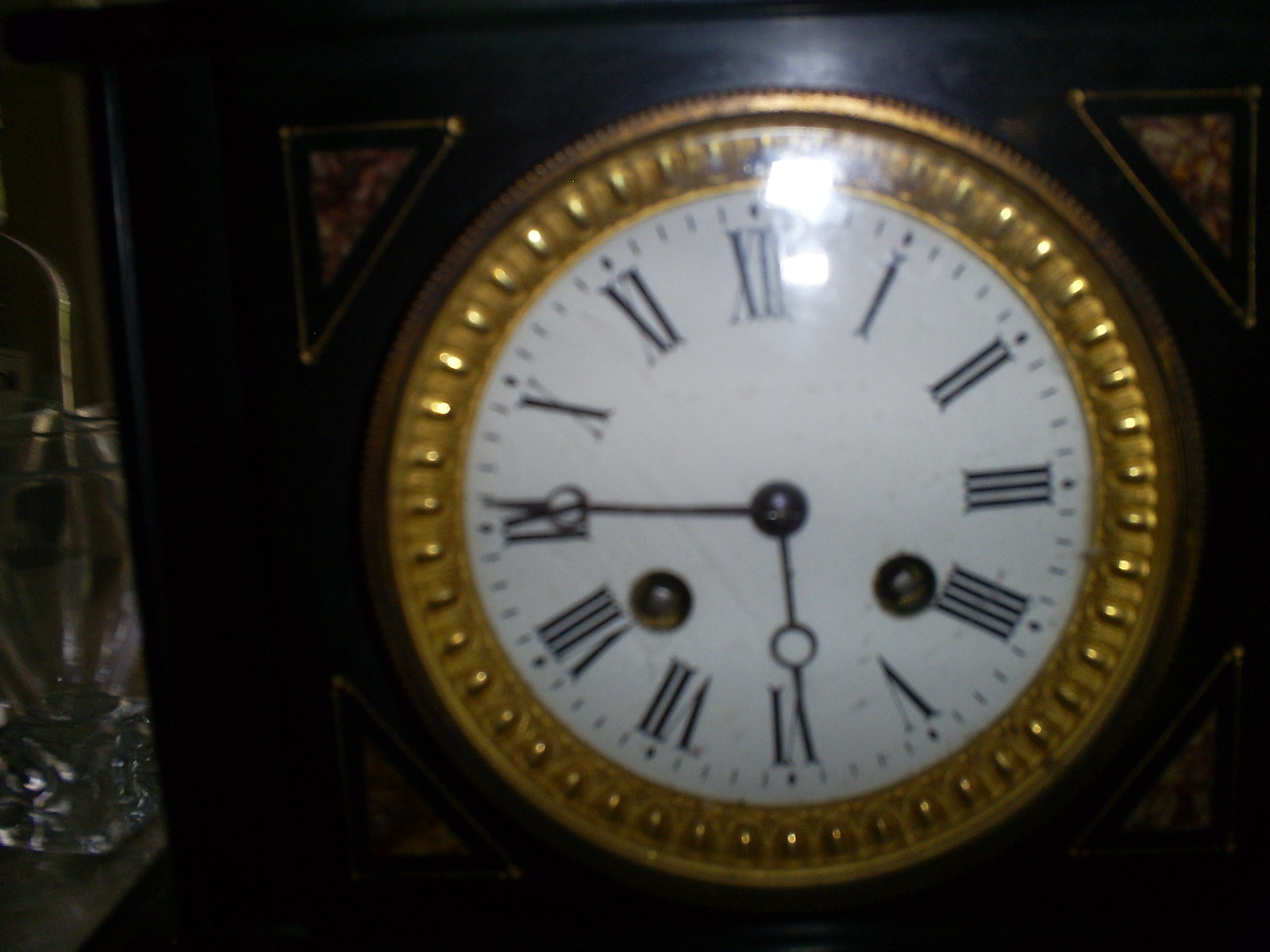This image features a clock with a round face encased in a square frame. The clock face is bordered with a gold-colored trim, contrasting elegantly with the dark brown, wooden frame. Notable are the small triangular shapes in each corner of the frame, each adorned with a multicolored design that adds an artistic flair. Instead of standard numbers, the clock face displays Roman numerals from I to XII, and it has two hands: a shorter one for the hours and a longer one for the minutes. To the left of the clock, a clear glass rests on a marble pedestal, providing a sophisticated touch to the scene.